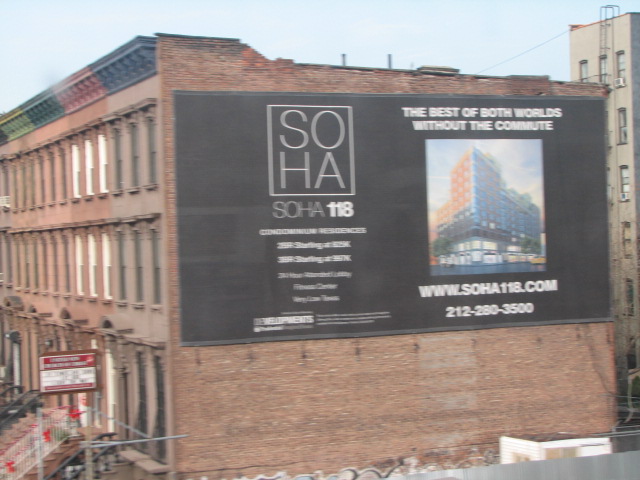The image depicts a weathered red brick building, viewed at an angle that reveals both its expansive side wall and a glimpse of its front facade. The building appears to be of historical or industrial significance due to its aged and somewhat crumbling exterior. The side of the building is adorned with a large black banner, which becomes the focal point of the image despite the center being slightly blurred.

The banner, with a black background, prominently displays the text "SOHA" twice, one above the other, in a white-rimmed outline. Below that, it reads “SOHA 118” in bold white lettering. Further down, in thinner white letters, it advertises "condominium residences" followed by details that become unreadable due to the blur. There is a high-rise artist's impression of the future project on the other half of the banner, suggesting the building's potential transformation. The tagline "the best of both worlds without the commutes" is visible, along with a website URL, www.soha118.com, and what appears to be an American phone number for inquiries.

The front facade, extending to the left edge of the image, exhibits a distinct architectural feature at the top—a multicolored section with hues of green, blue, red, and darker blue, contrasting the otherwise uniform red brick. The building spans three stories, including a potential basement level, with numerous windows dotting its length.

In the background, at the very right of the image, stands a tall, thin, beige building that appears to be five or six stories high, likely serving residential purposes. The sky looms above, casting light on the scene, and emphasizing the blend of old and new in this urban setting.

This promotional banner raises curiosity about whether the existing building itself is slated for renovation into the advertised condominiums, or if the advertisement refers to a nearby development project within the city.